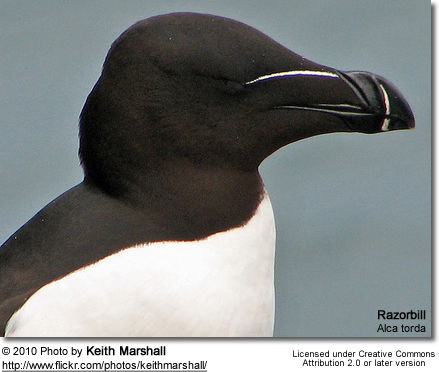The image features a striking side profile of a Razorbill (Alca torda) bird, set against a grayish background. The bird, predominantly black, showcases a sharply contrasting white chest. Notably, it has a distinctive white vertical stripe bisecting its otherwise black rounded beak, and a horizontal stripe extending from the beak towards its eye area, which appears either closed or nearly indiscernible due to the dark plumage. The bird is positioned on the left side of the frame, facing right, dominating the composition. In the bottom right corner, the text "Razorbill Alca torda" is written in small black letters, denoting its species. Below the image on the left side, the underlined text reads "© 2010 Photo by Keith Marshall," followed by the linked website "http://www.flickr.com/photos/keithmarshal." To the right, "Licensed under Creative Commons Attribution 2.0 or later version" is noted, signifying the photo's usage rights.